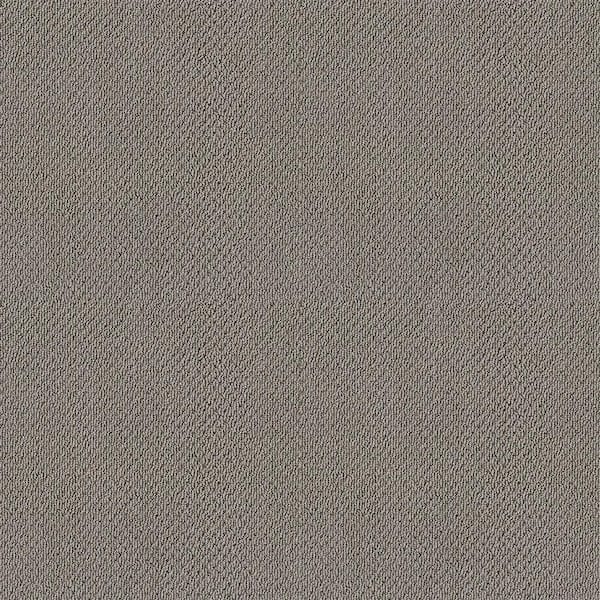This image depicts a square piece of woven fabric, likely photographed from above. The material appears to be designed for use as a rug, foot mat, or chair cover. The primary color of the fabric is a mixed shade of gray, interwoven with brown and possibly some greenish tints. Upon closer examination, darker threads or dots, potentially holes, are visible within the fabric, adding to its textured appearance. There might be a faint line or seam running down the middle, which may indicate a tear. Overall, this fabric possesses a slightly rough texture, and no other objects or text are present in the image.